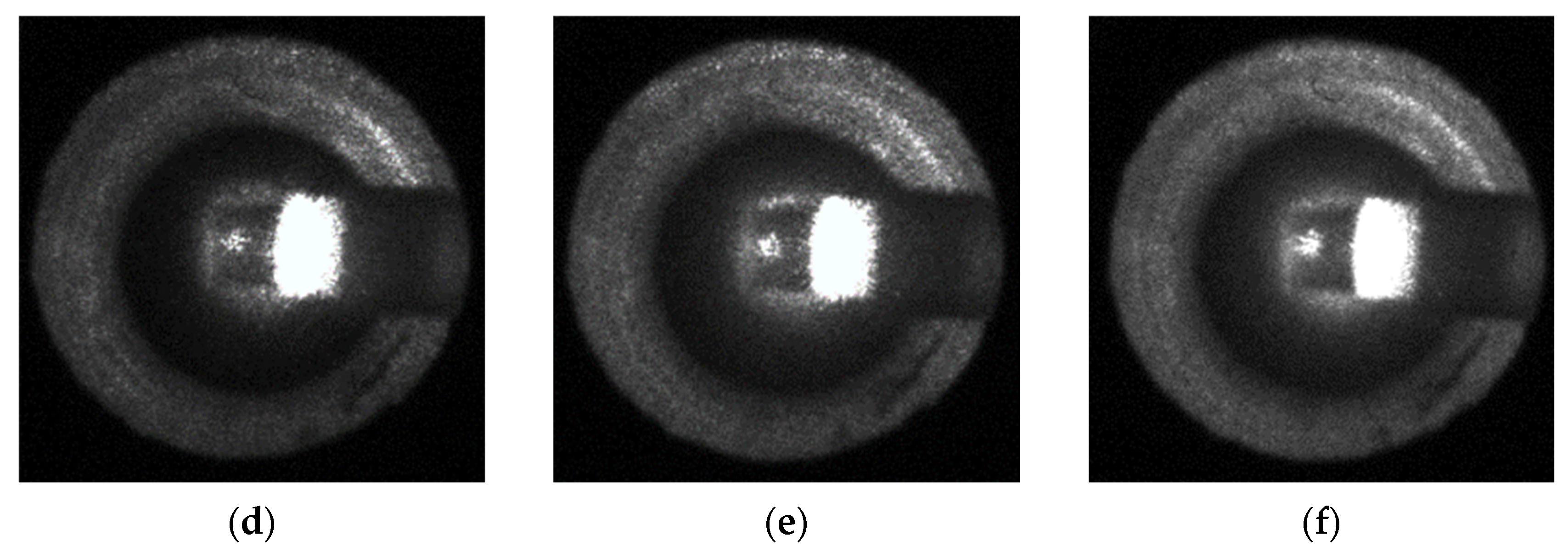The image appears to be a scientifically-oriented black and white collage consisting of three small circular images, each set against a black background. These circles resemble cells or microscopic structures, each with a central square-like lit area. From left to right, the images are labeled with letters D, E, and F in parentheses directly beneath them. The images are separated by a white border, creating a clear delineation between each. Despite slight variations in shape and size, all three circles share a similar dark and blurry texture, somewhat mimicking the view through a dim peephole. The overall visual is devoid of any other text or people, maintaining a focus on the circular shapes and their inherent glowing center.